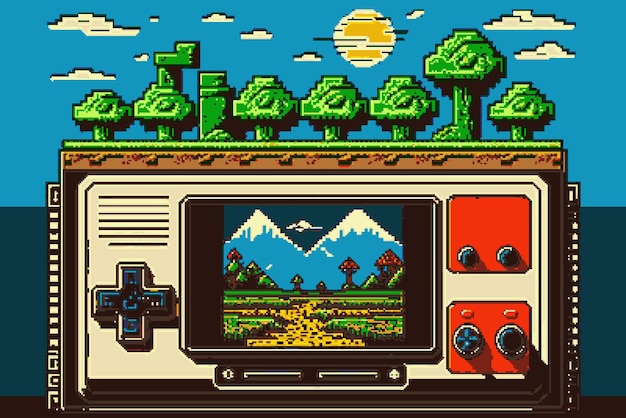This digital art piece vividly portrays a handheld Game Boy, rendered in white, with the iconic cross-shaped directional pad on the left and two action buttons on the right. Centered on the Game Boy's screen is a nostalgic scene reminiscent of classic video games, possibly inspired by the Mario Bros series. The in-game view features two white mountains in the background, framed by scattered clouds and a bright sun. In the foreground, there are large mushrooms, a dirt road leading toward the mountains, and additional paths branching left and right. Intriguingly, the Game Boy itself integrates into the environment with trees seemingly growing atop it. The artwork utilizes a color gradient in the background, with a dark blue hue at the bottom transitioning to a lighter blue towards the top, enriching the scene with depth and emphasizing the blend between the digital device and the vibrant, game-inspired world.